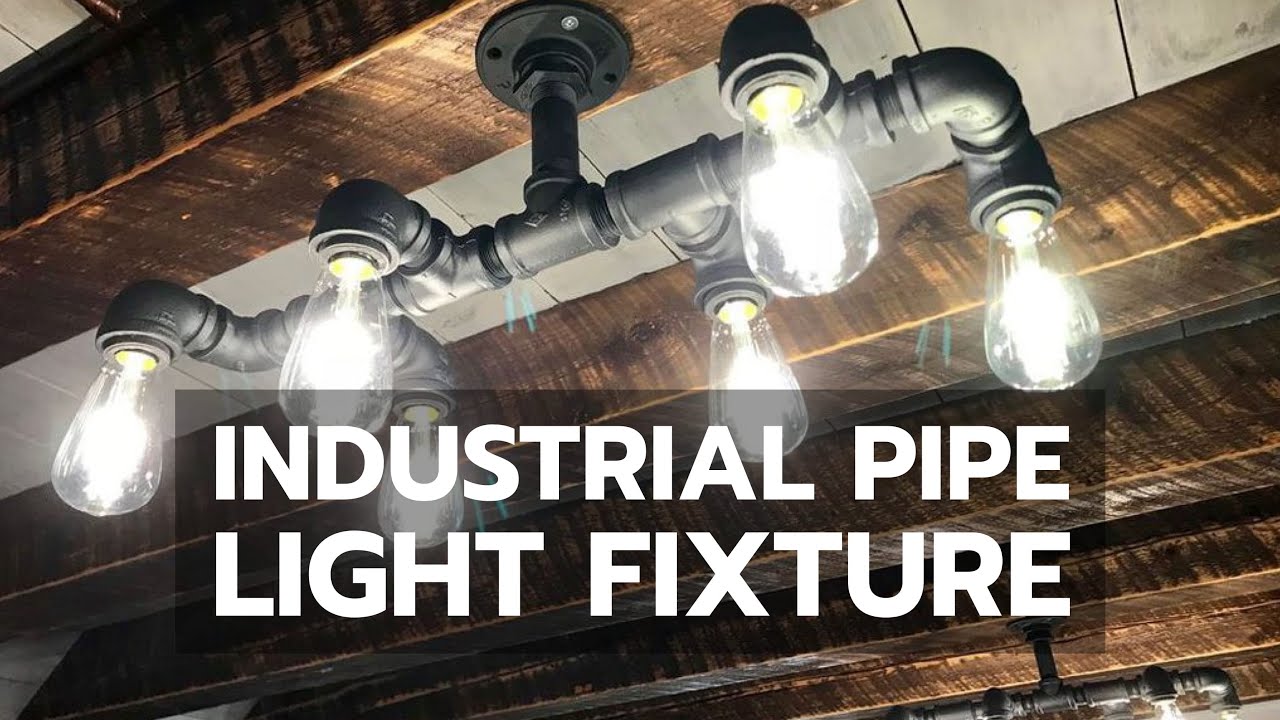The image depicts an industrial pipe light fixture, likely meant for an advertisement or as a product thumbnail. The fixture is elegantly designed with black metal pipes arranged in a non-symmetrical yet balanced fashion, extending out to six individual classic Edison bulbs, three on each side. Each bulb emits a bright white light, illuminating their vintage yellow bases. The background features a slightly transparent black opacity, allowing a detailed view of a rustic ceiling composed of weathered dark brown wooden beams and white-painted panels crisscrossing between them. The text "industrial pipe light fixture" is prominently displayed at the bottom in a clean white font, clearly conveying the product's theme.